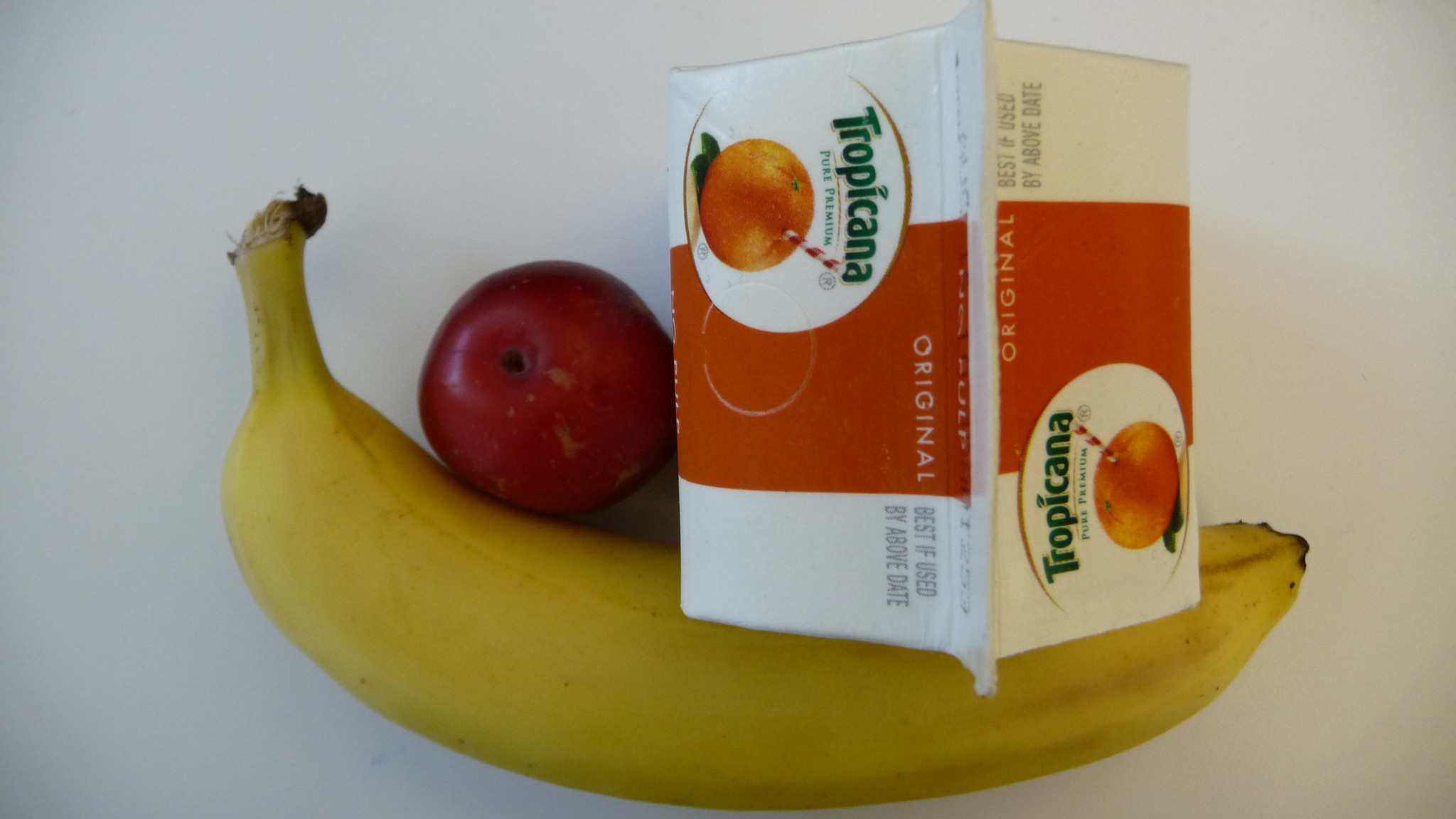In the center of the image, there is a slightly underripe yellow banana. Just above the banana is a stemless red apple. To the right of these fruits is a Tropicana Original branded orange juice container, designed to resemble a regular-sized milk carton. The carton is mainly white with an orange overlay, and the Tropicana logo is displayed in green. Above the logo, the carton features the phrase "Best if used by" although the exact date is not visible. The logo also includes an illustration of an orange with a red-and-white striped straw inserted. All items are placed on an unassuming white table. The lighting in the image is modest, suggesting it was taken in the early evening, around 5 to 7 p.m.